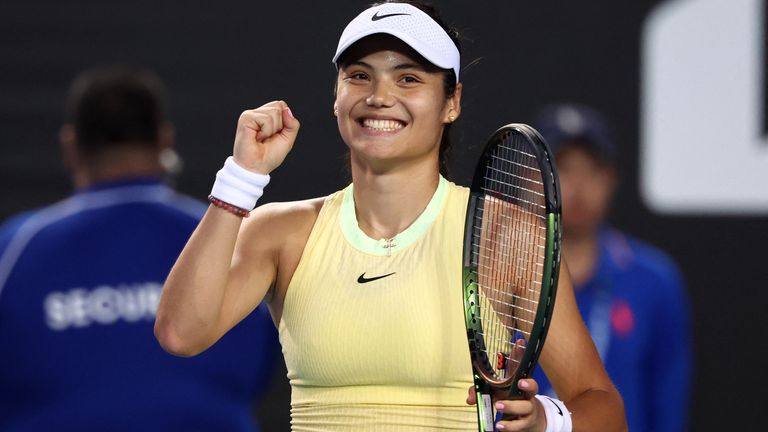The image is a professional photograph of a young woman, potentially of Hispanic, East Asian, or biracial descent, exuding happiness with a wide smile. She is holding a tennis racket with green and black rims in her left hand, while her right hand is clenched in a victorious fist. Dressed in a pale yellow, sleeveless Nike tank top and a white Nike ball cap, she also sports white sweatbands on both wrists, each emblazoned with the Nike logo; additionally, her right wrist bears a bracelet made of brown beads and a fresh pink manicure. The background is predominantly black, with two blurred figures behind her: one with a "Security" labeled dark blue jacket and another man in a blue jacket, possibly hinting at her recent triumph in a tennis tournament.